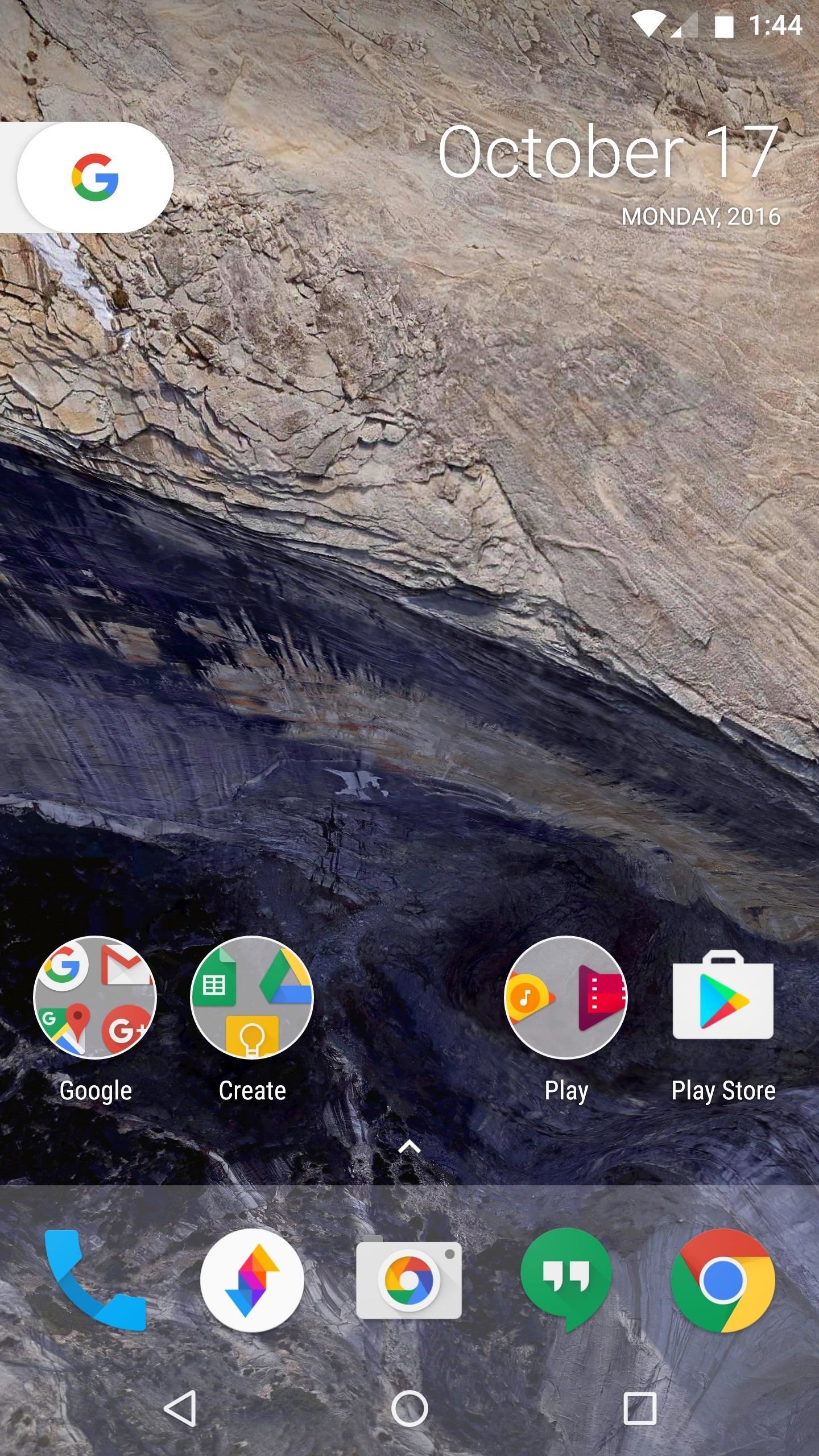In this screenshot of an Android device, we observe a detailed view of the home screen. At the top, the status bar displays several icons including the Wi-Fi icon, network signal strength indicator, battery level, and current time, which is 1:44. The date is shown as Monday, October 17th, 2016. Positioned at the top left corner is the Google search bar.

Moving towards the bottom of the screen, there are three clearly identifiable folders. The first folder contains a collection of Google apps: Gmail, Google Maps, Google+, and three additional Google applications. The second folder includes Google Drive among two other unnamed Google applications. The third folder houses Google Music and Google Movies apps.

Aside from the folders, the home screen also showcases individual icons for the Google Play Store, Phone app, Camera app, Hangouts, and Google Chrome, neatly arranged for easy access. The organized layout and selection of applications suggest a user who prioritizes Google services for their daily mobile needs.